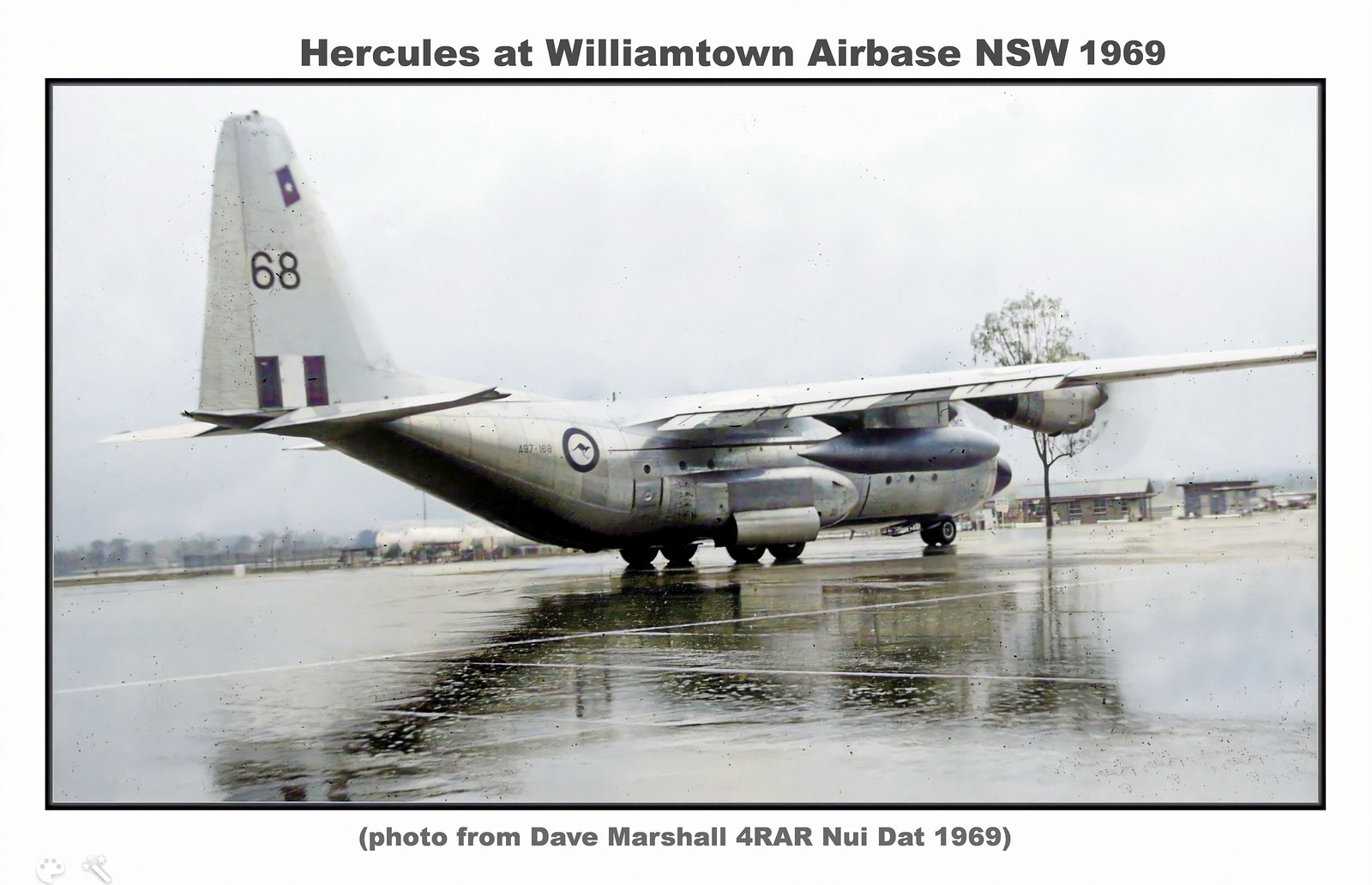The image depicts a silver Hercules transport airplane stationed at Williamtown Air Base, NSW in 1969. The photo, credited to Dave Marshall from 4 RAR Nui Dat, shows the plane facing right, with visible right-side wings and engine. The tail bears the number 68. The plane is parked on a slick, wet concrete area, indicating recent or ongoing rain. The background includes small buildings and a single tree to the right, with additional trees visible in the far distance on the left. The sky overhead appears cloudy and whitish, setting a somber, rainy day scene.